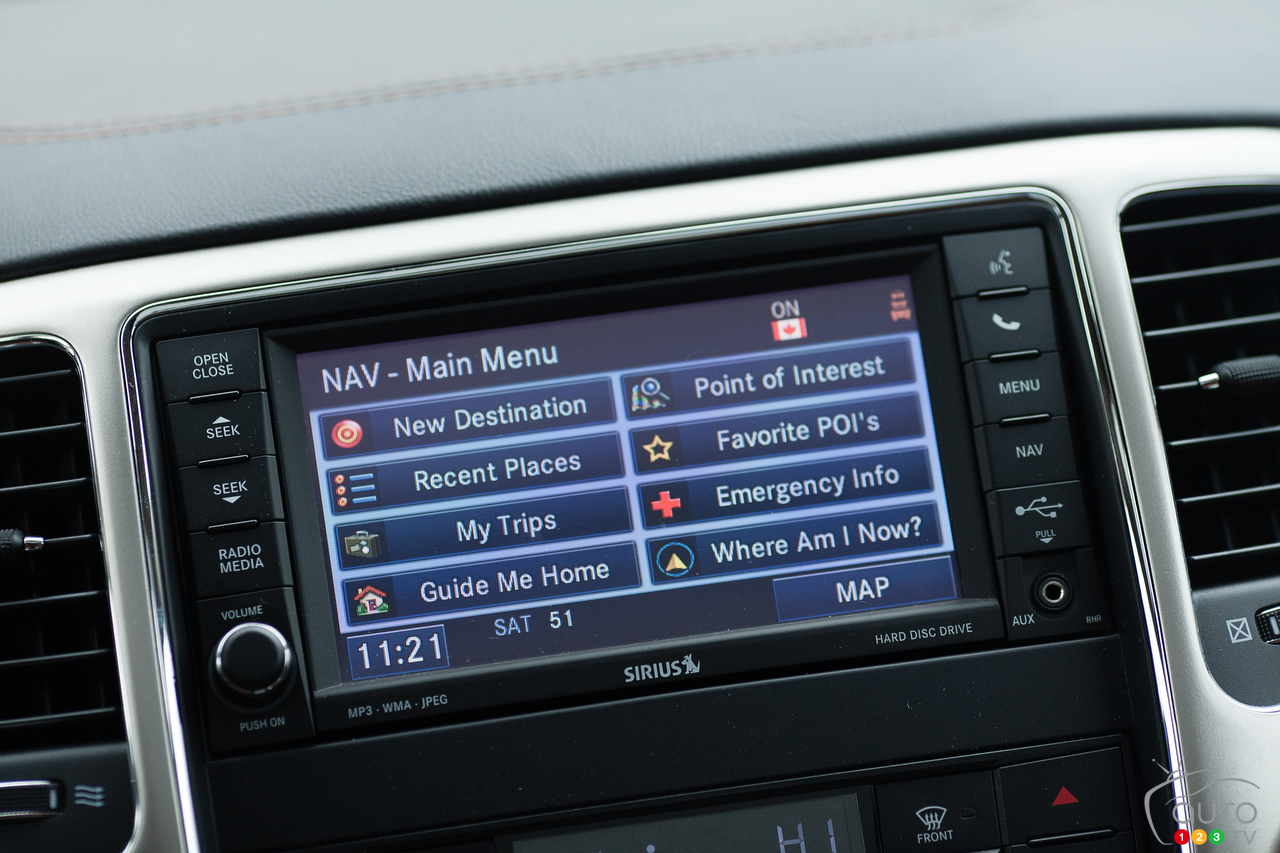The photograph depicts the center console of a car's dashboard, featuring a large, centrally-located multimedia system encased in silver trim and flanked by black air vents. Dominating the center is a widescreen LCD with multiple blue rectangular buttons. On the screen, the main menu options are displayed in light text against a dark background, indicating selections such as NAV, Main Menu, New Destination, and Point of Interest, organized into two columns. The first column includes options like Point of Interest, Favorite POIs, Emergency Info, and Where Am I Now. The second column lists New Destination, Recent Places, My Trips, and Guide Me Home. Below these options, the screen shows the current time, "1121," alongside a map. On the bezel surrounding the screen, the left side includes buttons for functions like Open, Close, Seek Up, Seek Down, Radio, Media, and a volume knob. The right side features buttons for Phones, Menu, Navigation, USB, and an AUX jack. At the top right corner of the screen, an "O-N" and a Canadian flag are visible, indicating the Sirius-brand navigation system.